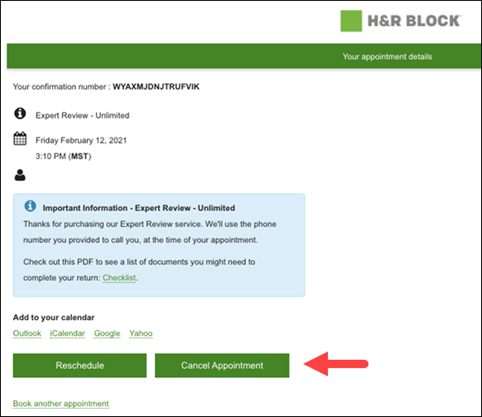The image is a screenshot from H&R Block's webpage detailing an upcoming tax appointment. A prominent green banner that spans the top of the page displays the appointment confirmation details. Notably, the appointment is confirmed with a lengthy alphanumeric code and labeled as "Expert Review Unlimited."

The appointment is scheduled for Friday, February 12th, 2021, at 3:10 p.m. Mountain Standard Time. There is a small calendar icon adjacent to the date and time. Additionally, a person icon is present, although it appears blank without specific information.

A blue information box, marked with a bolded title "Important Information," states: "Thanks for purchasing our expert review service. We'll use the phone number you provided to call you at the time of your appointment. Check out this PDF to see a list of documents you might need to complete your return." A clickable link to a checklist of necessary documents is provided.

The page also offers the option to add the appointment to various digital calendars, including Outlook, iCalendar, Google Calendar, and Yahoo. At the bottom, there are two buttons available for rescheduling or canceling the appointment, and a link to book an additional appointment if desired.